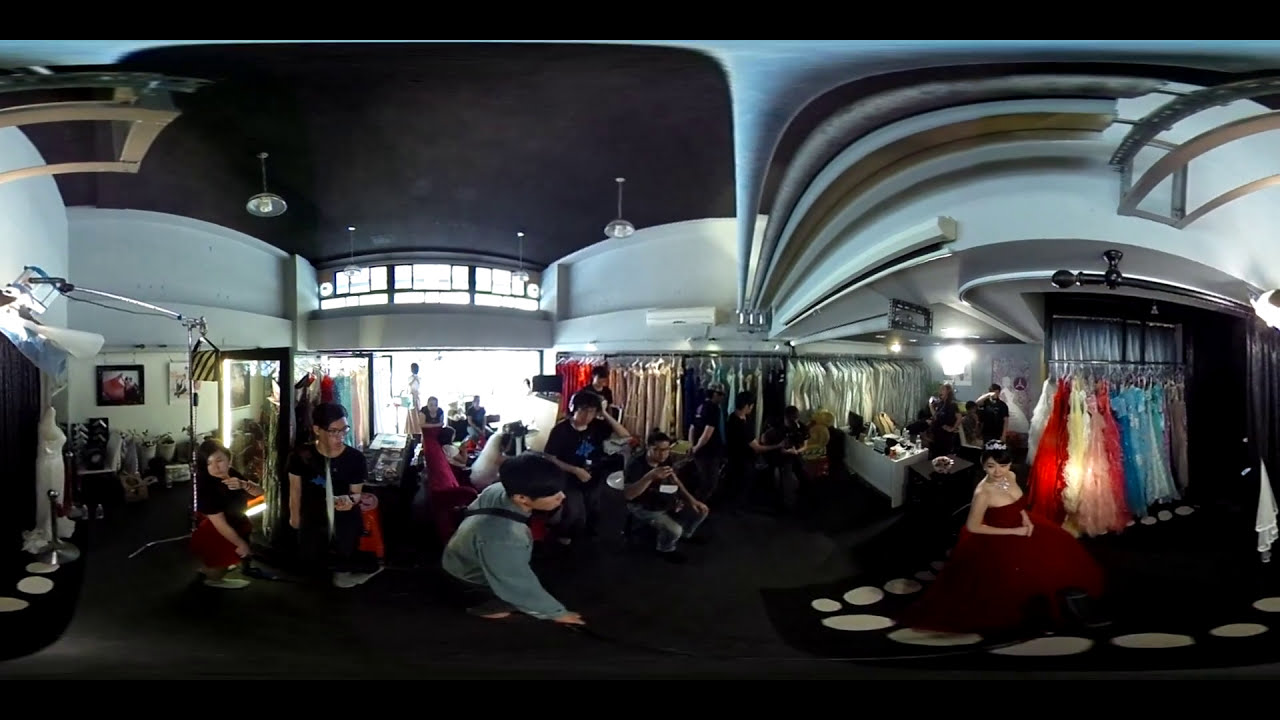The image captures the bustling interior of a backstage area, possibly at a fashion show or a theatrical event. The foreground features a young boy with dark hair wearing a long-sleeved grey t-shirt, only partially visible from the side. Centered in the image, a woman with black hair sits elegantly, adorned in a poofy, off-the-shoulder red gown with a tiara. She appears to be the focal point, surrounded by onlookers and various other individuals involved in different activities.

To the right of the image, a rack displays a variety of colorful gowns, including red, white, pink, light blue, and darker shades, organized likely by color. The scene is illuminated by fluorescent lights, while a window in the background reveals a lit street outside, adding natural light to the setting.

The ceiling, a hanger pattern with pipes colored blue, grey, brown, and white, contrasts against its blackish hue. Walls are painted white, contributing to the bright atmosphere. Makeup kits and models are scattered throughout the right side of the image, further enhancing the sense of backstage preparation.

Throughout the background, multiple people engage in various tasks, some standing next to organized racks of clothing. Each section of clothing appears color-coordinated, with distinct areas for beige, dark, and white outfits. A mannequin in a dress stands to the left, and a woman, seemingly looking over her shoulder, stands near a mirror, contributing to the dynamic and vibrant ambiance of this behind-the-scenes glimpse.